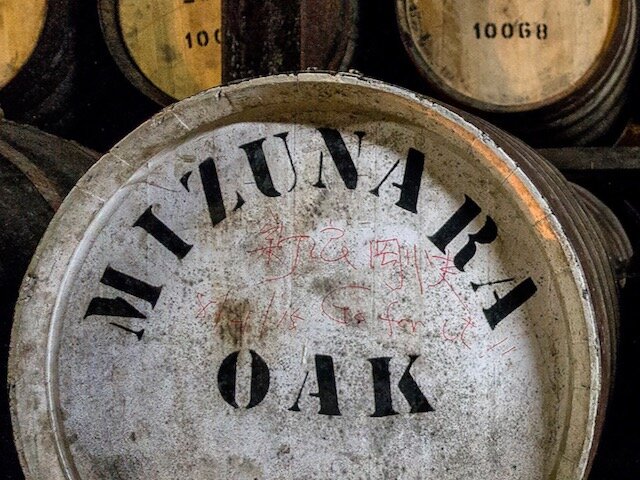The image captures a close-up of a wooden cask, primarily focusing on the end cap of the cask which is prominently displayed in the center. The cask is lying on its side, revealing a circular, weather-beaten, light-colored end cap. Stenciled in blocky, capital letters in an arched shape is the word "Mizunara," followed by the word "Oak" in a straighter alignment underneath. The letters appear hand-stenciled with slight misalignments. Between the words "Mizunara" and "Oak," there's faint, almost indiscernible Japanese writing in red ink. The sides of the cask exhibit a brown, wooden texture. In the background, partially cropped out, there are two other casks laid on a plank side by side, also showing their end caps. These background casks have a yellowish to tan tint and are labeled "100 G8." The overall scene provides a detailed, rustic look into the specifics of cask labeling and storage in what appears to be a whiskey or wine aging facility.